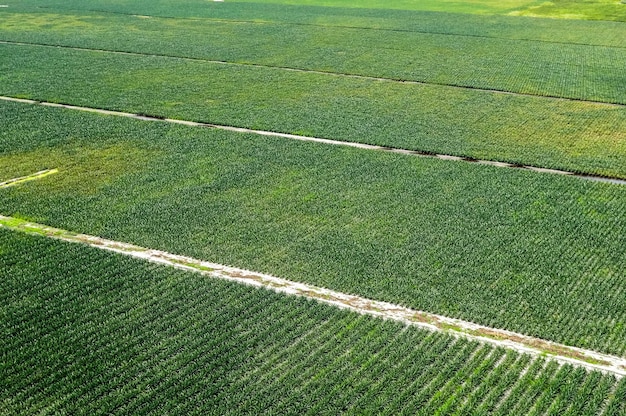This aerial image captures a detailed view of expansive farm fields, divided into six distinct sections by diagonal, grassy white gravel paths. The camera angle shows the fields from left to right, creating a dynamic perspective. The vibrant green fields, interspersed with rows of crops, appear leafy and verdant, possibly corn or soybeans, with some patches exhibiting a yellow-green hue. The white gravel paths intersect the fields diagonally, running from the upper left to the right-hand side, and another prominent white line extends from the middle left edge to the bottom right corner. The view is uninterrupted by irrigation systems, farming equipment, or people, highlighting the orderly, divided sections of thriving crops from an overhead vantage point.